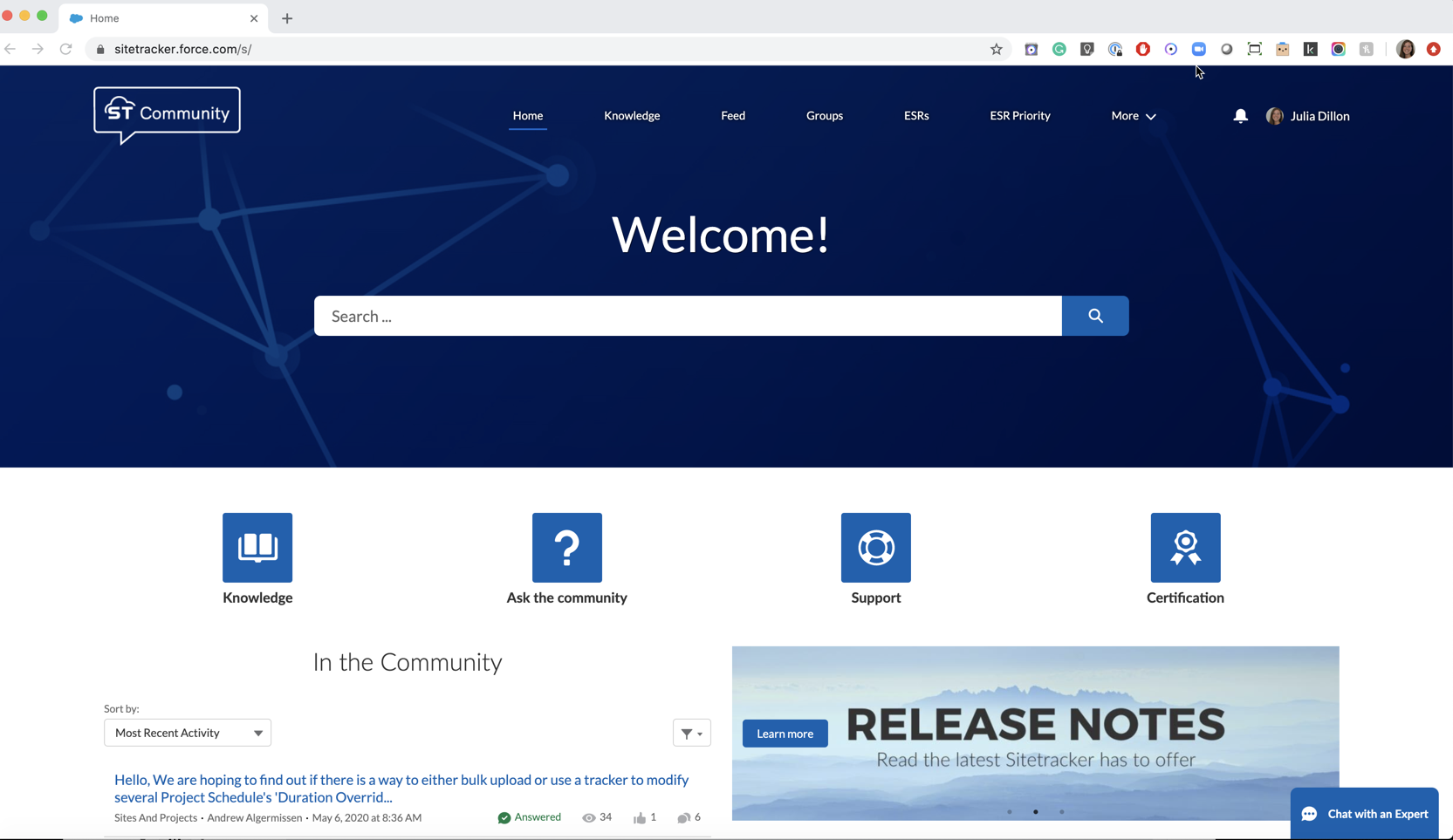The image depicts a computer screen displaying a webpage from the Site Tracker community on forest.com. The browser tab is labeled 'Home'. The webpage has a dark blue background adorned with geometric shapes that resemble a star map, with circles connected by straight lines. 

In the top left corner of the screen, a modified text box reads "ST Community" alongside the logo. The top navigation bar includes tabs labeled Home, Knowledge, Feed, Groups, ESRs, ESR Priority, a drop-down menu for more options, a bell icon for notifications, and a profile picture indicating that the user is currently Julia Dillon.

Prominently at the center of the screen, the word 'Welcome!' is displayed above a white search bar featuring a magnifying glass icon. Below this, a series of buttons are available for Knowledge, Ask the Community, Support, and Certification. The sidebar on the left includes an option to sort by the most recent activity, with the top listing displaying a message: "Hello. We are hoping to find out if there is a way to either bulk upload or use a tracker to modify several project schedules, duration, override."

Further down on the left side, there is an image promoting 'Release Notes', inviting users to 'Read the latest Site Tracker has to offer' with a button to 'Learn More'. Finally, in the bottom right corner, a blue bar offers the option to 'Chat with an Expert'.